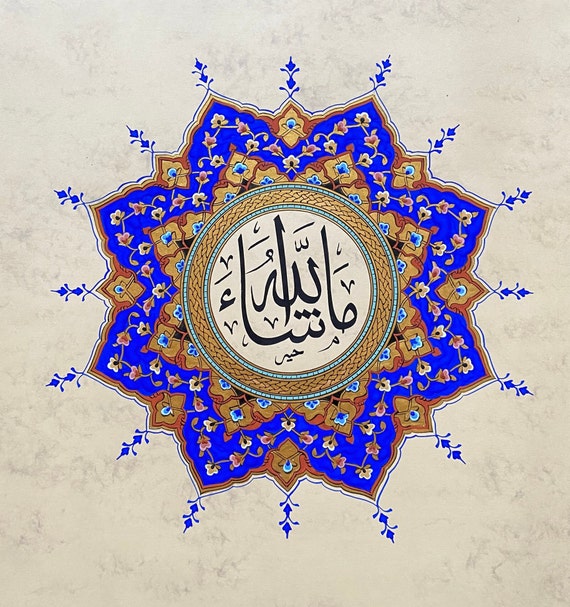The image features a highly detailed, computer-generated Middle Eastern-inspired symbol set against a light tan, marbled background with some gray spots. Dominating the center is an elaborate star-like shape with approximately twenty triangular points. The star is bordered in brown and filled with bright blue, eye-catching shading. At each of the star’s points, blue stems sprout with attached leaves, enhancing the visual appeal. Encircling the star's central area is a tan circle adorned with black characters resembling a Middle Eastern script, enclosed by a thick, darker brown braided pattern. The overall composition is colorful and animated, incorporating various shades of blue and brown, along with a discernible, zigzag leaf pattern within the bright blue areas of the star's border, adding to the intricate and vibrant design.